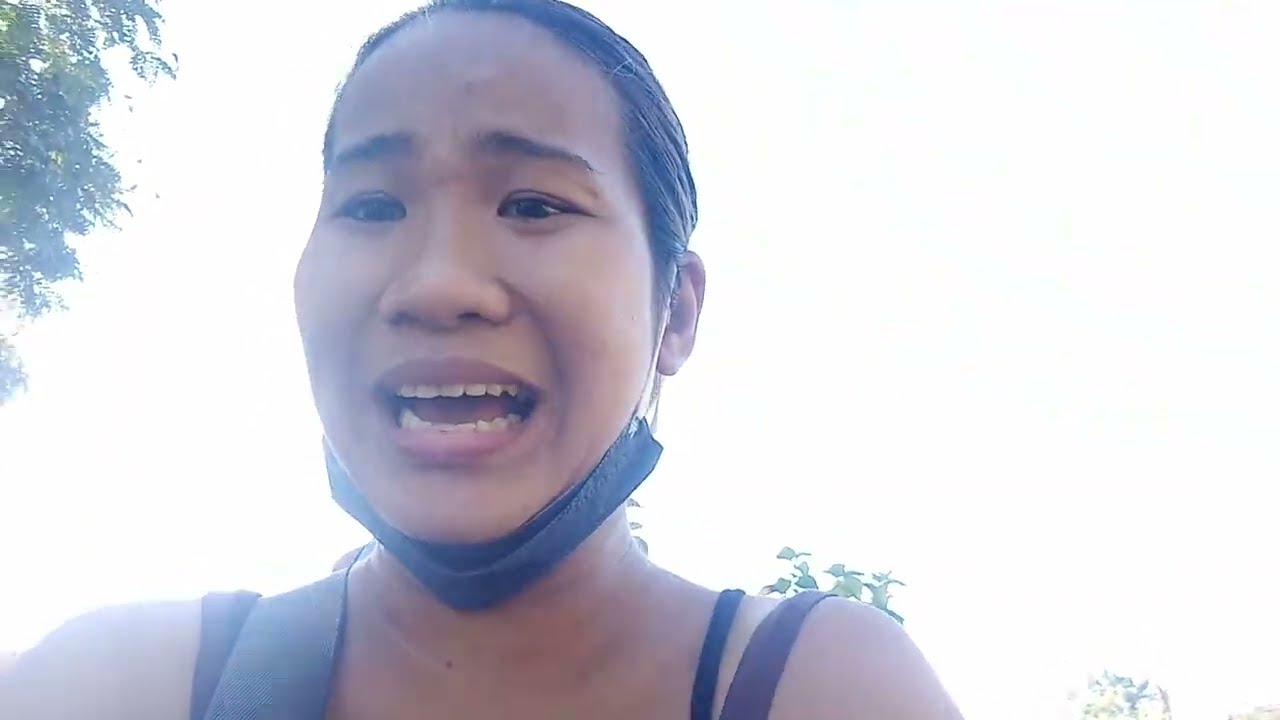An image of a distressed Asian woman, captured from the shoulders up, is set against a brightly lit background. Her hair is pulled back tightly into a ponytail or bun, exposing her fearful eyes and open mouth, as if she is crying out. She is wearing a black spaghetti strap tank top, complemented by what appears to be a wider strap, possibly from a bag or camera, across her left shoulder. A dark-colored surgical mask with white ear loops is pulled down under her chin, revealing both rows of her teeth. The background is predominantly bright, making it difficult to distinguish details, but there are visible green leaves from trees in the upper left and lower right corners of the image. The overall scene conveys a sense of distress and anxiety.